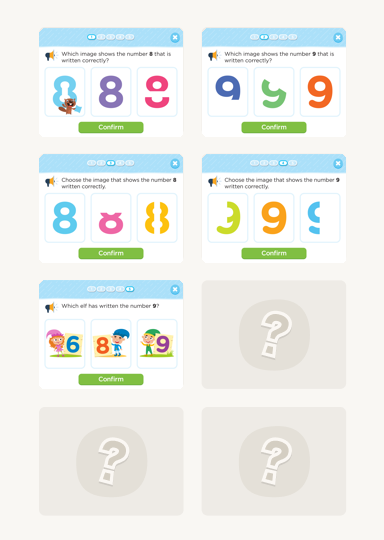The image is a screenshot from an educational app designed for children to help them learn how to correctly recognize and select numbers. The interface features multiple pictorial questions where kids are asked to identify the correct representation of a number among three options. For example, the screen displays three variations of the number 8, two of which are drawn incorrectly and one that is accurate. Similar questions are repeated with numbers 8 and 9.

The app includes charming characters such as little elves and a brown raccoon, which likely serve to engage young users. The layout incorporates elements that appeal to children, such as multicolored numbers in pink, blue, purple, and green. Additionally, some areas of the screen feature blank question marks, hinting at interactive elements or upcoming questions.

Overall, this engaging and colorful app uses playful graphics and familiar characters to make learning numbers an enjoyable activity for children.